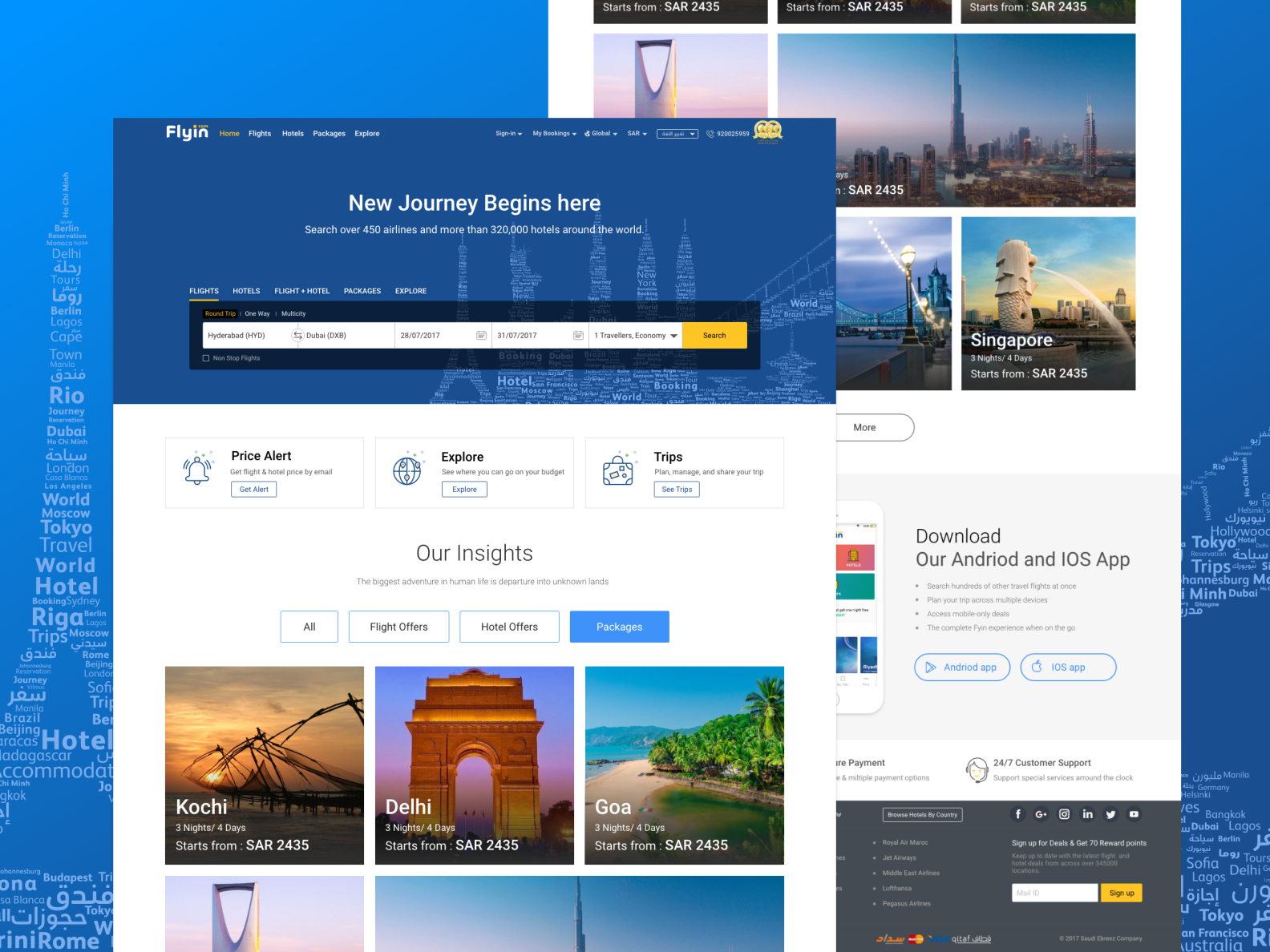This detailed caption provides a polished and vivid description of the screenshot:

---

This image is a screenshot of a travel agency's web page with multiple layers in its design. The background features two distinct halves. On the left, a blue section displays a word cloud forming the shape of an iconic structure resembling the Eiffel Tower, with names of various places in white text. The right section showcases square images promoting different vacation destinations, accompanied by a call-to-action to download the agency’s Android and iOS apps, along with additional information about the website.

In the foreground and slightly to the left, a highlighted section catches the eye with a blue label reading "Fly-In" in white text. This section is part of the main navigation bar with the menu options: Home, Flights, Hotels, Packages, and Explore. To the right of these options, there are buttons labeled Sign In, My Bookings, Global, three unreadable options, and a gold emblem.

Below the navigation bar, a prominent banner states "New journey begins here," inviting users to search across over 450 airlines and more than 320,000 hotels worldwide. Directly beneath this banner is a search bar offering categories for Flights, Hotels, Flight + Hotel, Packages, and Explore. 

Further down, there are sections titled Price Alerts, Explore, and Trips. The segment following these features "Our Insights" on a white background, with filter options for All, Flight Offers, Hotel Offers, and Packages. The Packages category is selected, displaying fully visible package deals for Kochi, Delhi, Mumbai, and Goa.

---

This well-structured caption provides an organized and comprehensive snapshot of the web page, making it easy to visualize the layout and content.